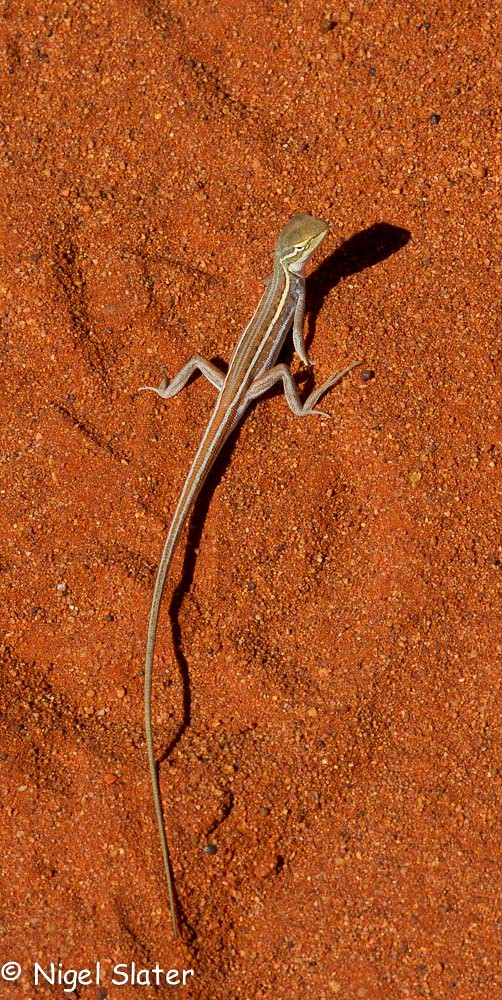In this photo, a small, slender lizard is captured on a very bright orange and red dirt background resembling a desert landscape. The ground appears to be a mix of fine sand and small rocks. The lizard, which is quite skinny with a needle-like, extremely long tail, is positioned in a way that makes it seem as though it is posing for the camera. The reptile’s body is adorned with brown and white colors, featuring two yellow stripes down each side of its back, with hints of green and orange. The lizard is primarily on its hind legs, with visible shadows of its head and body cast on the ground. A copyright notice with the name "Nigel Slater" is prominently displayed in the bottom left corner of the image.